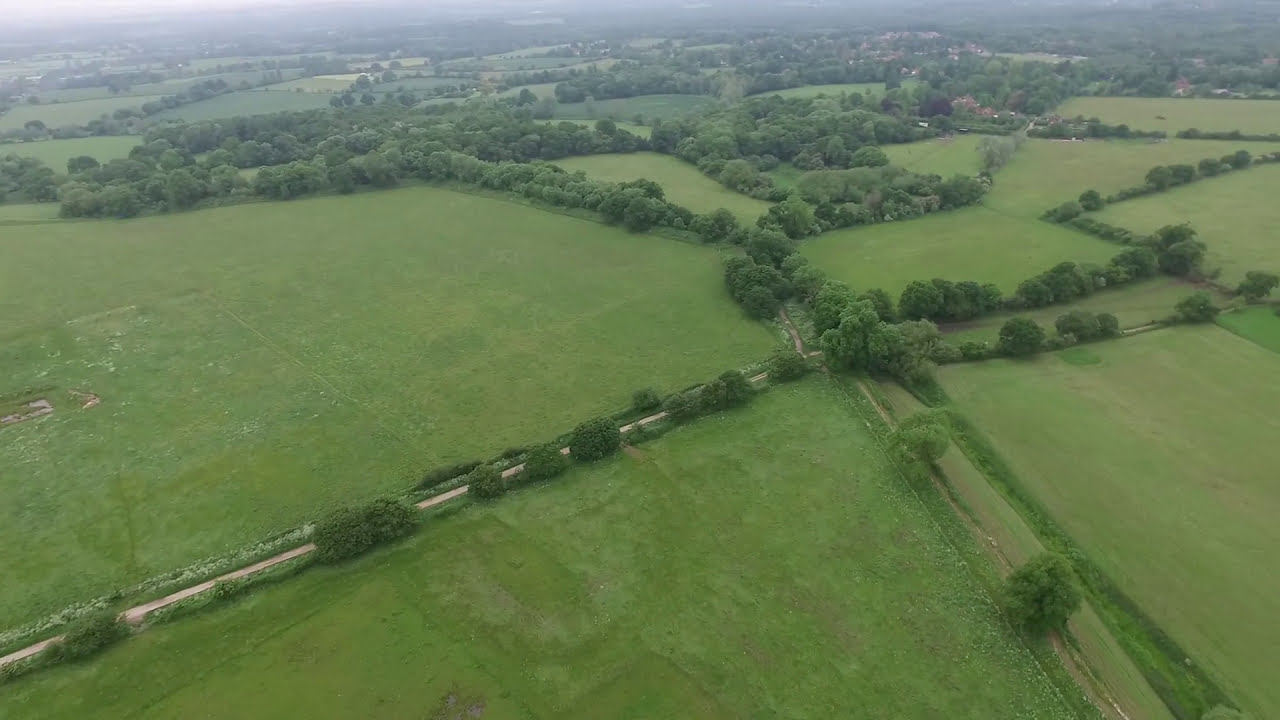This color photograph, captured by a drone, offers a breathtaking bird's eye view of a sprawling rural landscape during the middle of the day. The composition is predominantly dominated by large, open grassy fields in various shades of green, interspersed with rows of rounded trees. A road starts from the lower left corner, winding towards the center of the image before diverging into less distinguishable paths. Towards the top of the image, there is a denser concentration of trees and several small buildings, indicative of a modest settlement. The horizon in the distance gives off a hazy, blueish hue, with the upper left side appearing slightly lighter, suggesting the direction of the sunlight. The overall scene is realistic, accurately depicting the serene and expansive nature of the countryside.